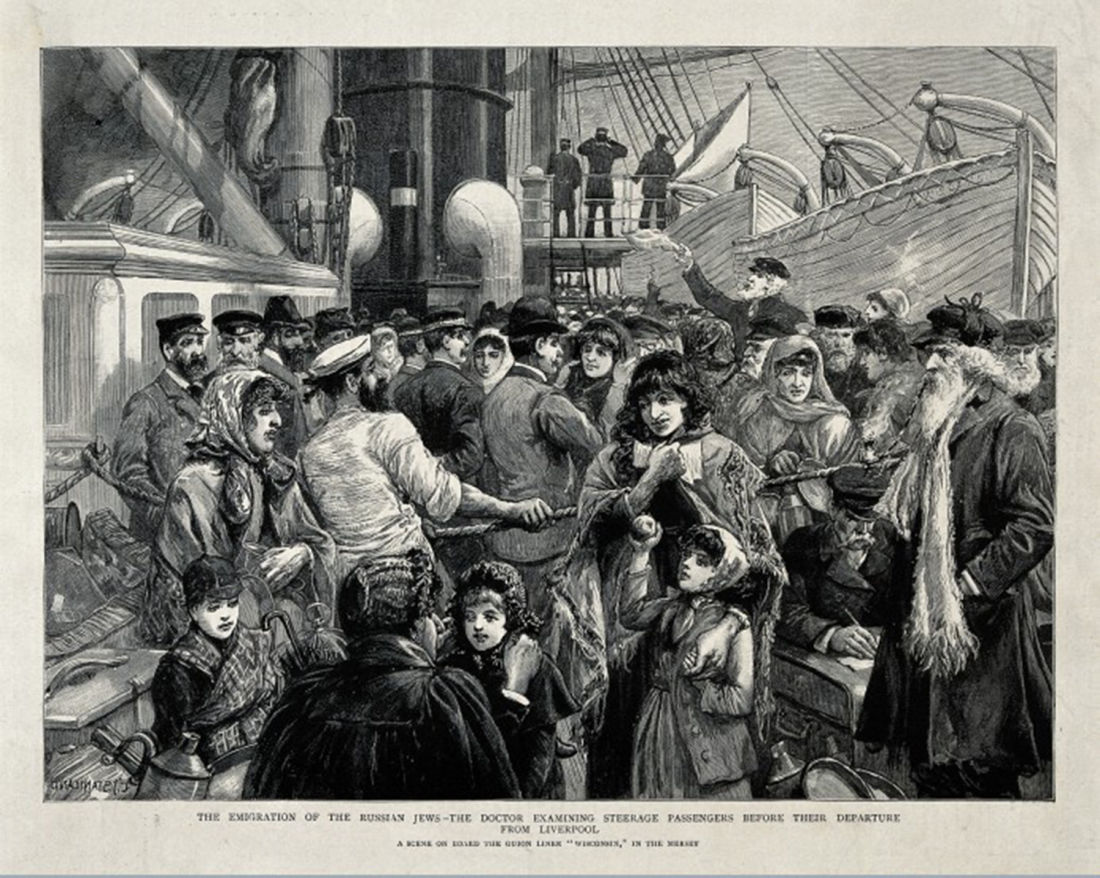The black and white etching depicts a crowded scene of Russian Jewish immigrants preparing for departure from Liverpool. The image captures a Victorian-era steam vessel, bustling with activity on both the dock and the ship. In the foreground, an elderly woman with a bonnet kneels, comforting a young girl, while a little boy and another girl stand close by. Nearby, a sailor in a white hat pulls a rope, possibly docking the vessel. The crowd includes people of all ages, dressed in poor, peasant-like clothing typical of the late 1800s to early 1900s. Men with long, scraggly beards and women with bonnets or scarves cover their heads. Above, lifeboats are hoisted, and a white flag flutters in the top right quadrant. There is text at the bottom stating, "The Immigration of Russian Jews — the doctor examining steerage passengers before their departure from Liverpool," with additional, unreadable smaller text beneath.